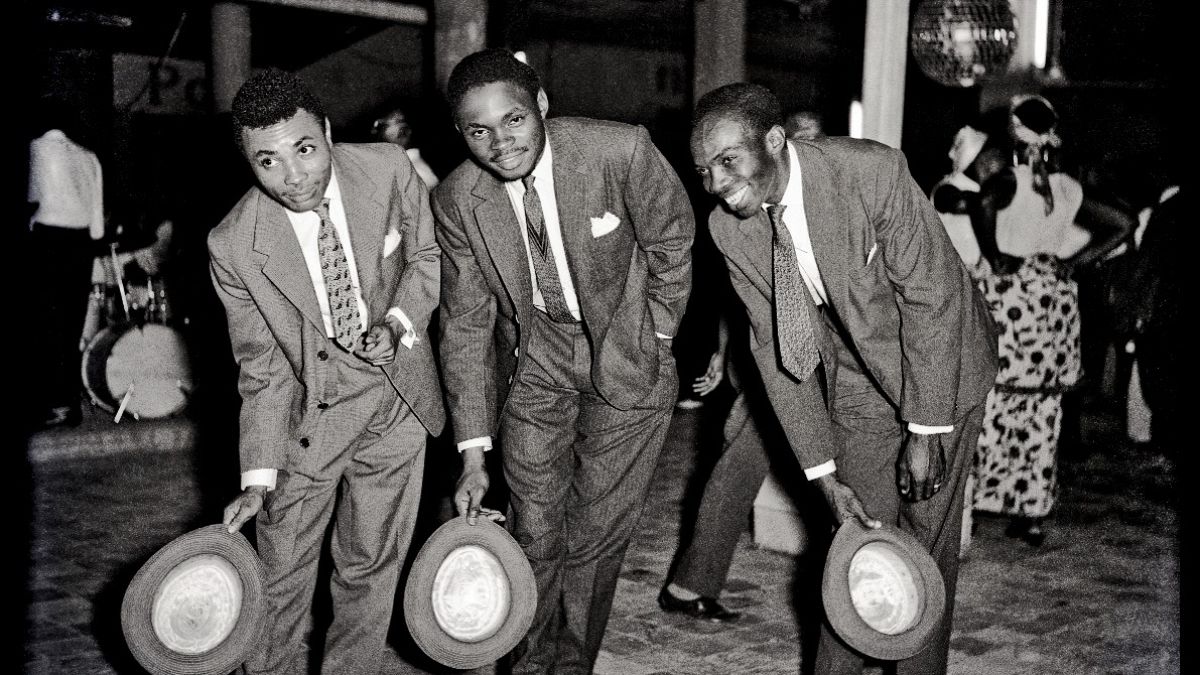In this black and white photograph, three men dressed in suits are the central focus, each holding a hat in their left hand, bent slightly forward. The man on the left wears a top hat, the one in the middle holds a fedora, and the man on the right also has a top hat. These men, possibly in their 40s or 50s, have pocket squares and are posing with smiles; the man on the right is smiling broadly, while the other two have more reserved expressions. The background, dimly lit, reveals a drum set on the left, suggesting a musical setting, possibly a club or a dance hall, featuring a disco ball overhead and tiled or carpeted flooring. Various indistinct figures, including what appears to be a waiter or band members, populate the backdrop, adding a lively yet subdued ambiance to the scene.